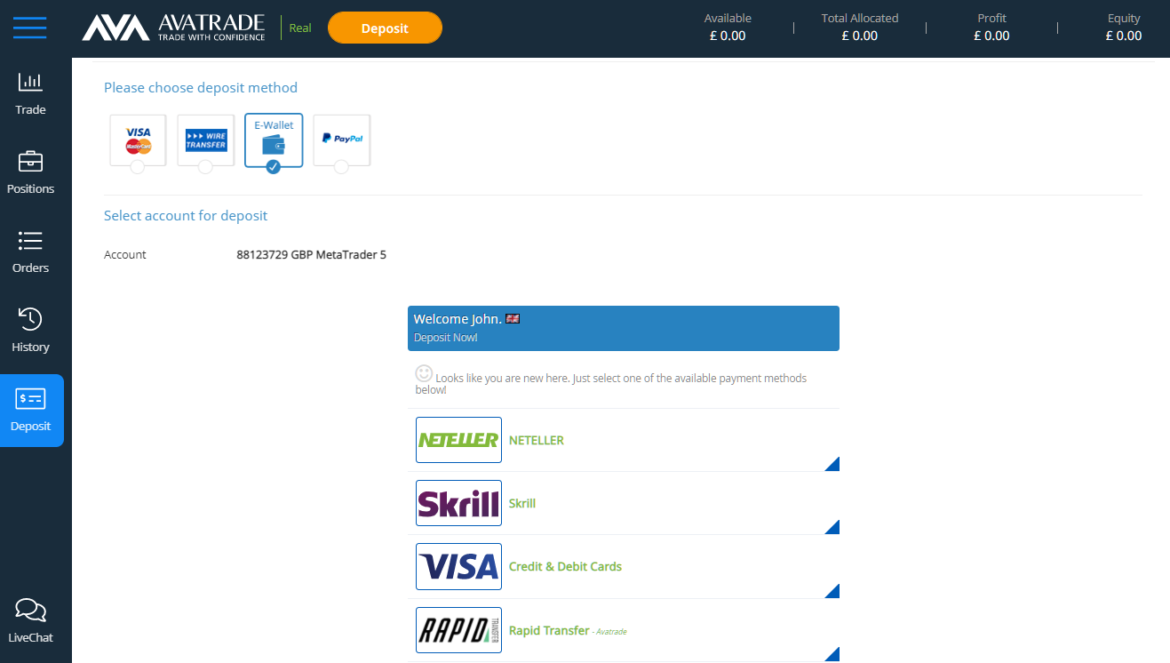Screenshot Description: Detailed View of AvaTrade's Trading Platform Dashboard

The screenshot captures the backend dashboard interface of a trading website, specifically AvaTrade. Dominating the top portion of the screen is a sleek black bar that runs horizontally across the page. Positioned on the top left of this bar is the AvaTrade logo, which is composed of three triangles – two pointing upwards and one in the middle pointing downwards. Accompanying the logo is the tagline, "Trade with confidence."

Adjacent to this, a vertical black sidebar is located on the left side of the screen. This sidebar features key navigational buttons labeled as Trade, Positions, Orders, History, and Deposit. These options provide users with easy access to various functionalities and sections of the trading platform.

Central to the page, a prominent white box contains a user prompt saying, "Please choose deposit method." Below this prompt are listed several payment methods, including Visa, Bank Transfer, eWallet, and PayPal, each presumably represented by their respective icons. Further down, there is an instruction to "Select account for deposit," suggesting that users can specify the account into which they wish to deposit funds.

Overall, the interface combines a blend of intuitive navigation and essential financial functionalities designed to enhance user experience on the AvaTrade platform.